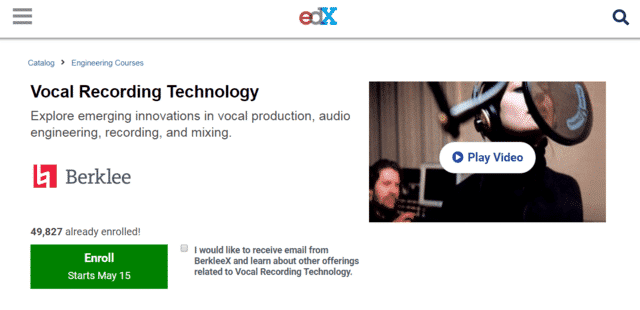Screenshot of the edX Website Featuring Berklee's Vocal Recording Technology Course:

The screenshot showcases the homepage of the edX website, which is similar in branding to FedEx but without the "F." At the top right side of the interface, there's a search button, while the top left side features a menu icon with three horizontal lines, indicating a drop-down menu option.

Immediately below the main navigation bar is the course catalog section. Displayed prominently is the text "Catalog Engineer Courses," followed by the course title "Vocal Recording Technology." A descriptive subheading invites users to "Explore Emerging Innovations in Vocal Production, Audio Engineering, Recording, and Mixing."

To the right of this text is an image depicting a woman in a professional recording studio, singing into a microphone. Standing behind a mixing console in the background, a man is seen adjusting the recording settings. The image includes a "Play Video" button, suggesting that a video related to the course can be viewed.

Underneath the image, the caption states that "49,827 already enrolled" in the course, with the enrollment starting on May 15th. 

Below this information, there's a checkbox option that reads, "I would like to receive emails from Berklee X and learn about other offerings related to vocal recording technology."

This detailed description captures the essence of the page and the various elements that it contains, providing a comprehensive overview of the course offering from Berklee on the edX platform.